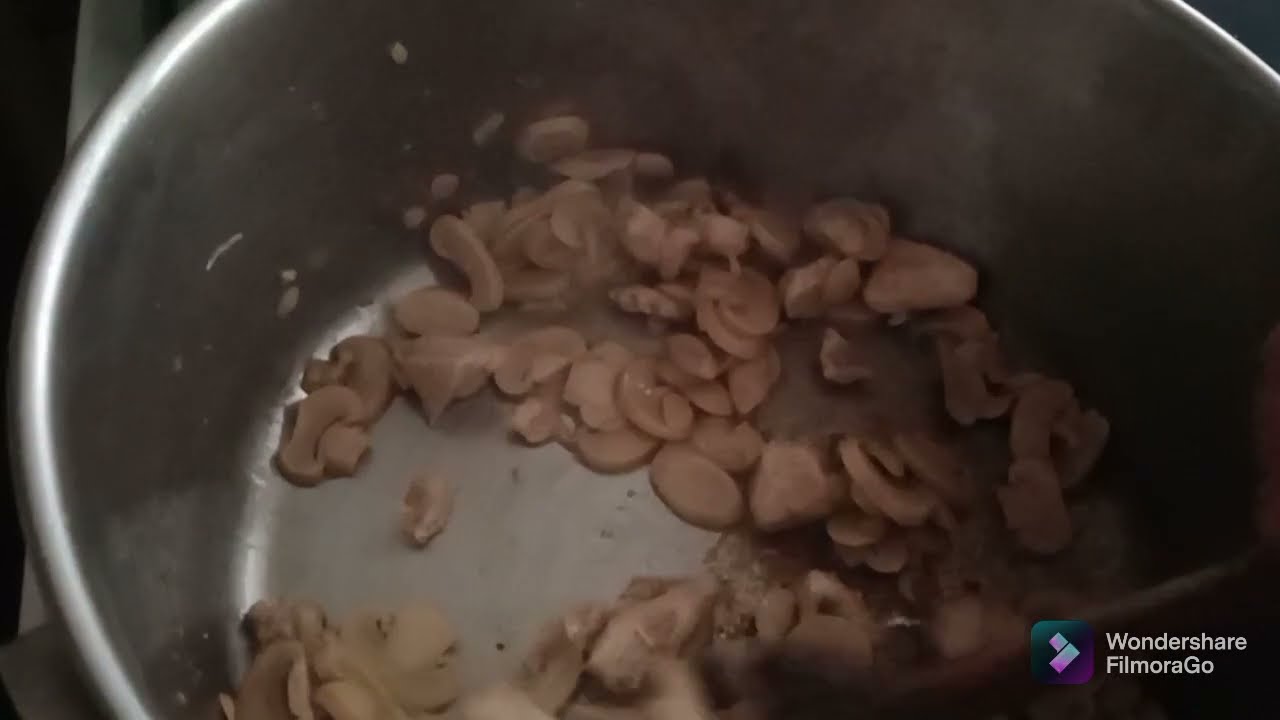This image features a close-up perspective as if one is leaning over and looking down into a metallic gray, possibly silver mixing bowl. Inside the bowl, sliced mushrooms, thin and almost slivered, are visible, suggesting they are being prepared or sautéed. The lighting, possibly from daylight or a well-lit room, reflects off the top edge of the bowl, highlighting the shiny surface. The majority of the background is dominated by the bowl, with blurred black and silver streaks appearing behind it. On the bottom right corner of the image, there is a logo, which includes the text "Wondershare FilmoraGo." This logo comprises white text and an accompanying teal, purple, and black icon with arrow symbols.